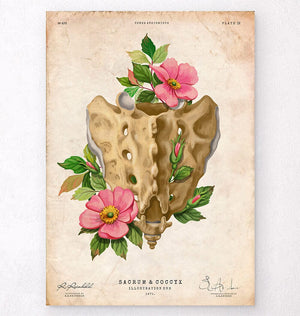The image is an illustrated picture resembling old parchment paper with an off-white, slightly cracked and browning appearance. At the top center and top left and right corners, there is very small black text that is difficult to decipher, with additional text at the very bottom and to the left and right edges, some of which is in cursive. The prominent text in the center reads as "Sacrima Gogi X" or something similar, though this is also somewhat unclear. The main illustration features a tan, bone-like structure with multiple holes, possibly resembling a vertebra, from which two pink flowers with yellow centers and surrounding greenery are growing. The image carries a shabby chic aesthetic with pale pinks and brown edges, evoking the feel of an old, delicate, and beautiful card or poster.